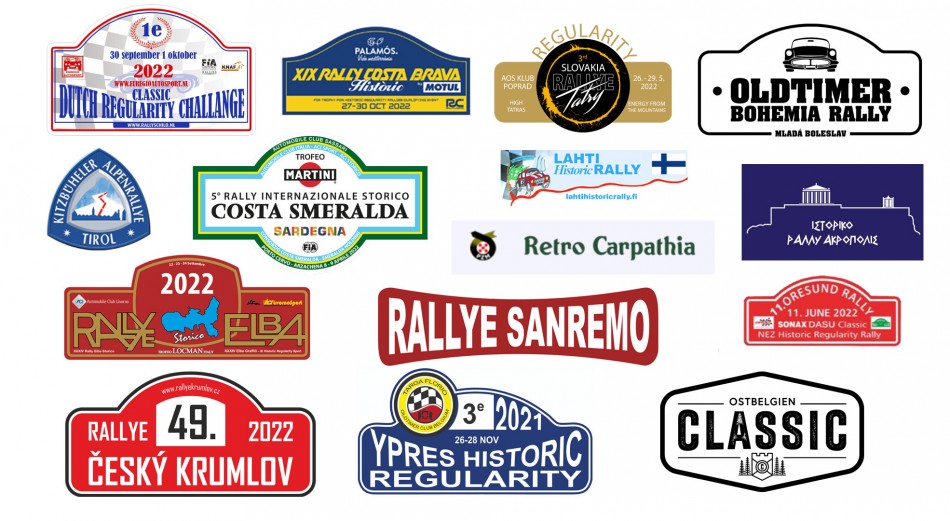This image showcases a vibrant collection of 15 distinct logos, primarily for various car rallies and races from around the world. The logos vary widely in style and color, representing events from different years and countries. Notably visible are the 2022 Dutch Regularity Challenge, the 2019 Rally Costa Brava Historic, Regularity Slovakia, and the Old-timer Bohemia Rally. There are also logos in different languages, including one in Greek and another for the Costa Smeralda Rally. Additional mentions include the Finland rally featuring its flag, the 2022 Rally Elba, and the Rally San Remo. The colorful assortment also features logos for the Retro Carpathia, Laity Historic Rally, and the Kitzbühel Alpenrallye Tyrol. This diverse array suggests a collection of bumper stickers or memorabilia from various international road rallies, appealing to enthusiasts who celebrate their participation in these events.